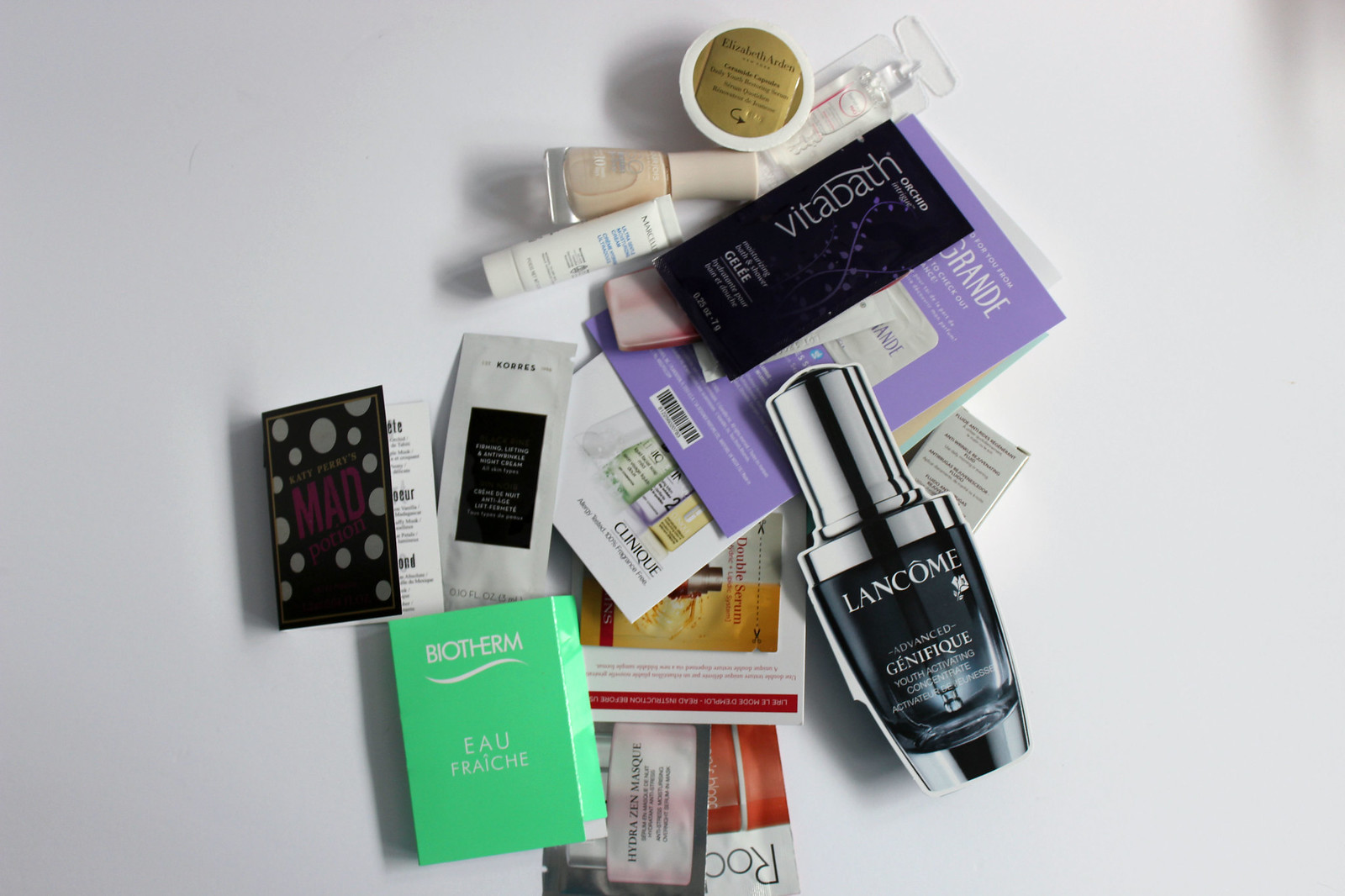The image portrays an assortment of health and beauty aid samples meticulously arranged against a bluish-white backdrop. In the bottom left corner, a green sample labeled "Biotherm Eau Fraiche" stands out, indicating a French perfume product. Adjacent to it lies another perfume sample, "Katy Perry’s Mad Love," featuring a distinctive black cover adorned with white spherical accents. 

Moving to the right, a collection of serum samples catches the eye, including a prominent "Lancome Advanced Genifique" with its sleek black bottle and silver lid. Scattered among these are small tubes of lip products, one notably white with a screw-top lid. Adding to the variety are makeup items; a glass bottle with a neutral-colored lid sits towards the upper part of the arrangement, potentially containing nail polish or concealer, given its neutral hue.

Each item is carefully positioned to showcase a diverse range of beauty products, creating a vibrant and inviting display.